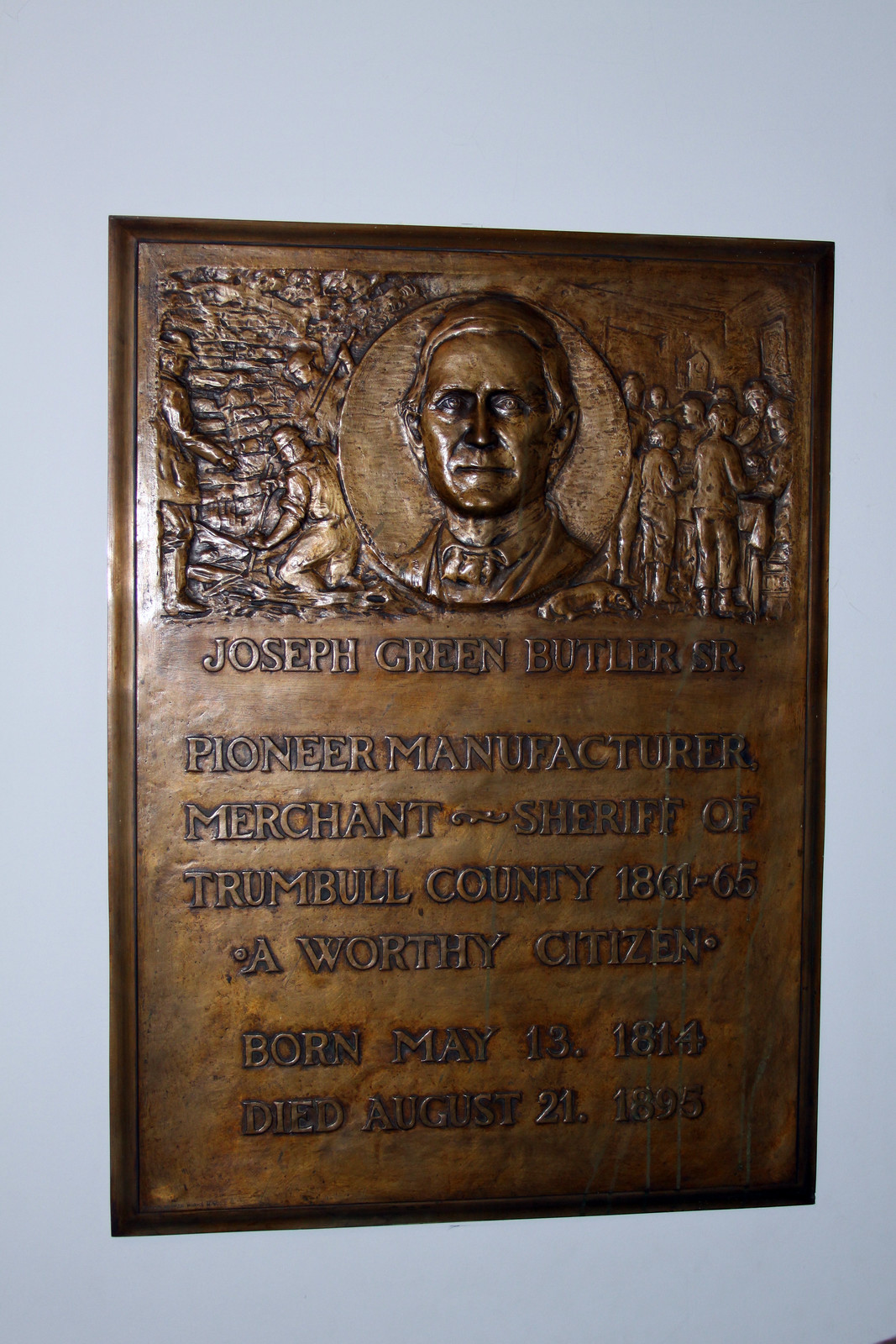The image depicts a detailed bronze memorial plaque affixed to a wall. The plaque features an engraving that is divided into several distinct sections. In the top left half, there are intricate reliefs of three men, possibly miners or soldiers, engaged in a laborious task of digging or striking, their sculpted forms capturing the essence of their effort. To the top right, a scene with up to ten engraved children appears, suggesting an indoor setting and adding a sense of historical narrative to the artwork. Central to the piece is a prominent bust of a man, etched meticulously into the bronze. Beneath this portrait is an inscription that reads: "Joseph Green Butler, Senior. Pioneer Manufacturer, Merchant, Sheriff of Trumbull County, 1861-1865, a worthy citizen. Born May 13, 1814. Died August 21, 1895." The plaque, rich in detail and craftsmanship, serves as a tribute to Joseph Green Butler, Senior, celebrating his contributions and legacy.